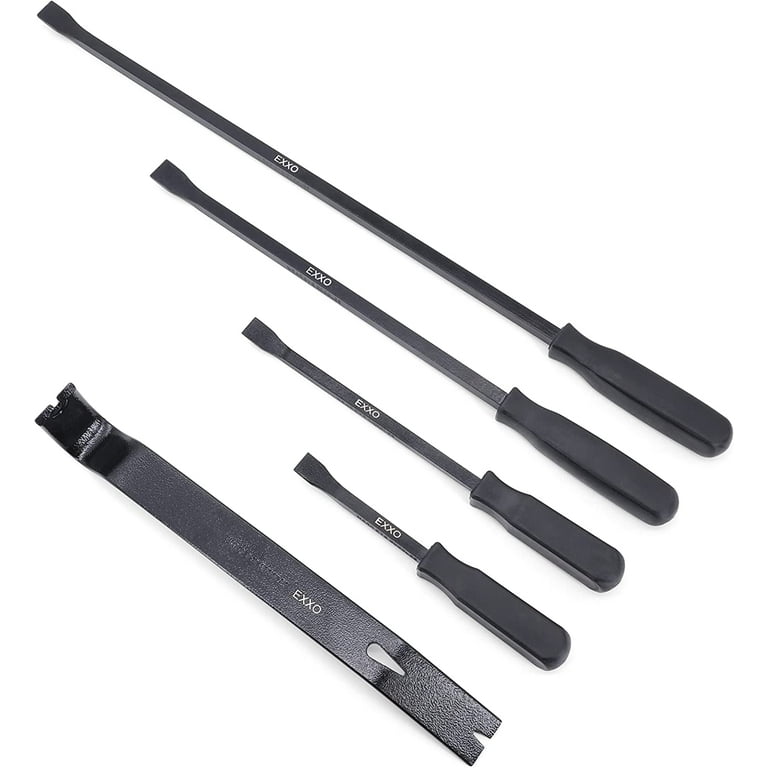The image showcases a set of five specialty tools, all inscribed with the letters "XO" in white on their central locations. The tools are arranged diagonally from the bottom left to the upper right. The tool at the bottom is a crowbar with "XO" engraved on it, featuring flat notches at both ends, resembling a pry bar. Above it, there are four similarly designed tools with black handles akin to screwdrivers, each with a progressively longer metal rod culminating in angled, chisel-like tips. These tools seem tailored for precision tasks like opening containers. The crowbar, as well as these four tools, all prominently display the "XO" marking at the midpoint of their metal shafts.